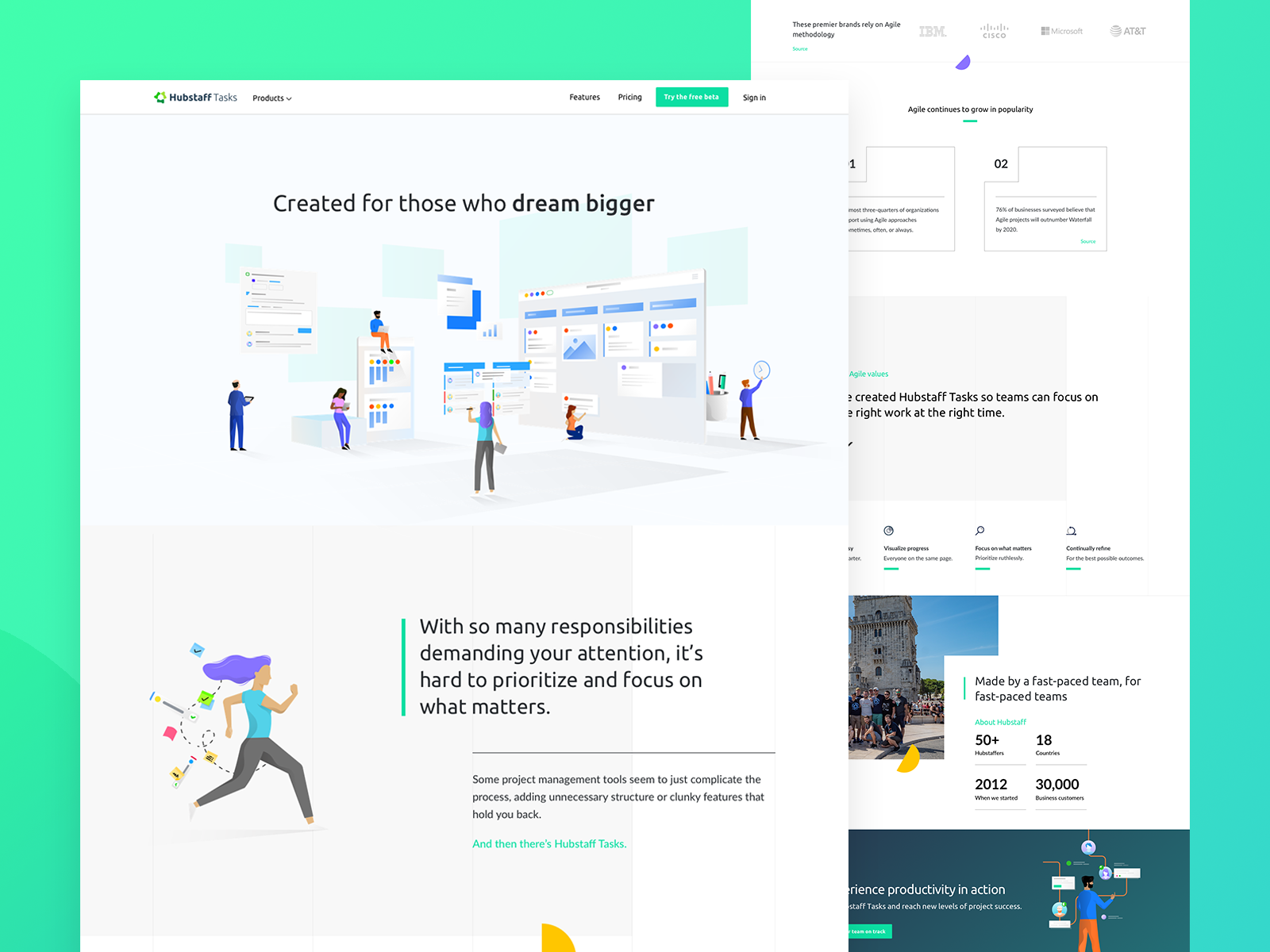The image features a webpage with a green border and a white background. At the top of the page, there is a navigation bar with the following options: Help, Staff, Task, Products, Features, Pricing, and Sign-in. In bold black lettering, a headline states, "Creative for those who dream bigger". 

Beneath this headline, there is an illustration of six cartoon characters, with drawings of computer screens and other tech-related imagery behind them. Below the characters, a subheading reads, "With so many responsibilities demanding your attention, it's hard to prioritize and focus on what matters." 

To the left, there is a cartoon character with purple hair, wearing a bluish short-sleeve shirt and black pants, depicted in a running pose. Further down the page, another block of text states, "Some project management tools seem to just complicate the process, adding unnecessary structure or clunky features that hold you back."

To the right, there is another section with a white background that says, "These premier brands rely on agility methodology." At the bottom of this section, there is an image showing a large group of people standing in front of a building, with a blue sky background. Adjacent to this image, a statement reads, "Made by a fast-paced team for fast-paced teams."